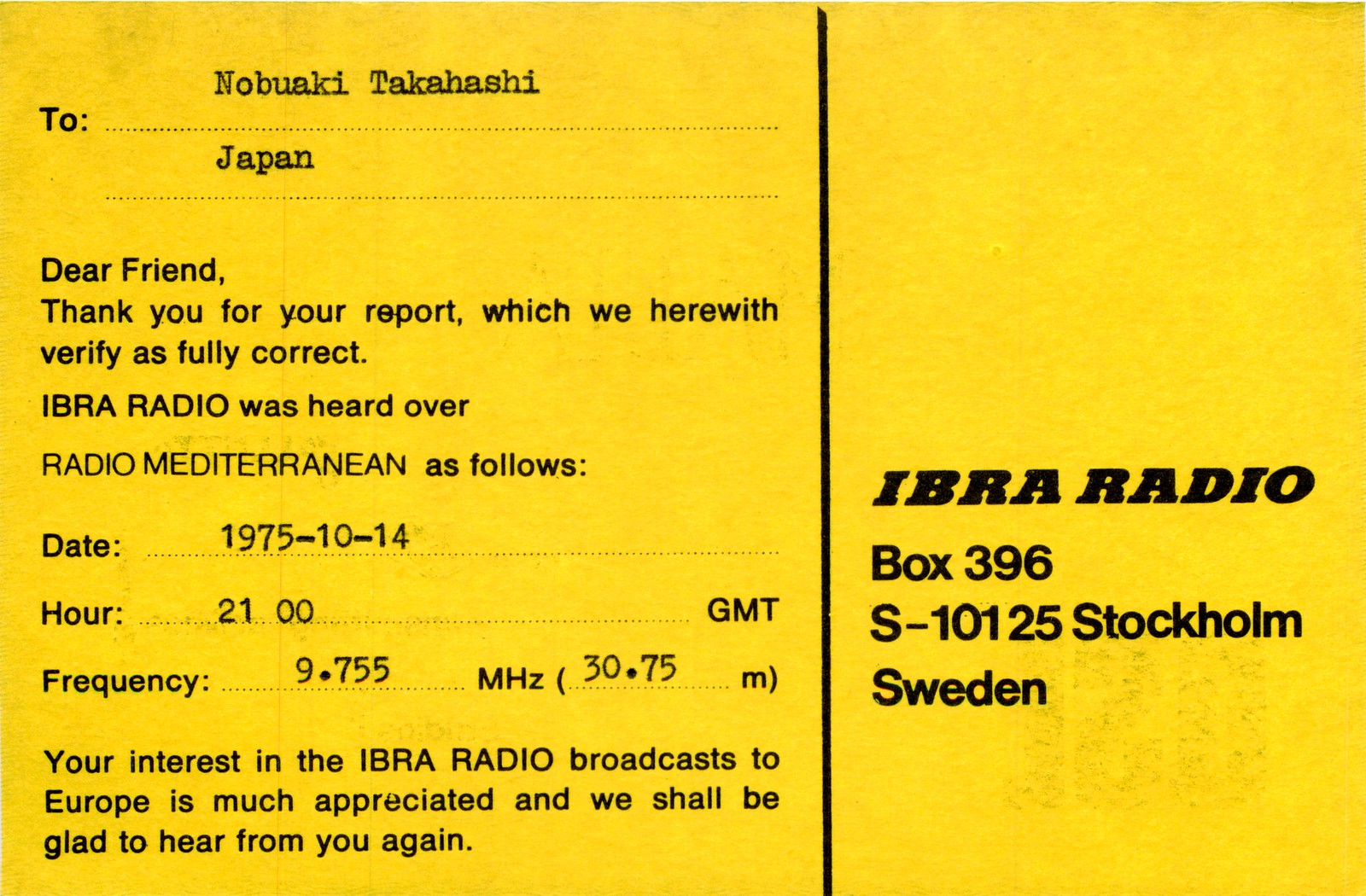This image depicts a vintage postcard from 1975 with a yellow background. In the center, slightly to the right, there is a distinct vertical black line. To the left of this line, the postcard is addressed to Nobuaki Takahashi in Japan. The text reads: "Dear friend, thank you for your report, which we herewith verify as fully correct. IBRA Radio was heard over Radio Mediterranean as follows: date 1975-10-14, hour 2100 GMT, frequency 9.755 MHz (30.75 M). Your interest in the IBRA Radio broadcasts to Europe is much appreciated, and we shall be glad to hear from you again." On the right side of the vertical line, the address is listed as "IBRA Radio, Box 396, S-10125, Stockholm, Sweden."